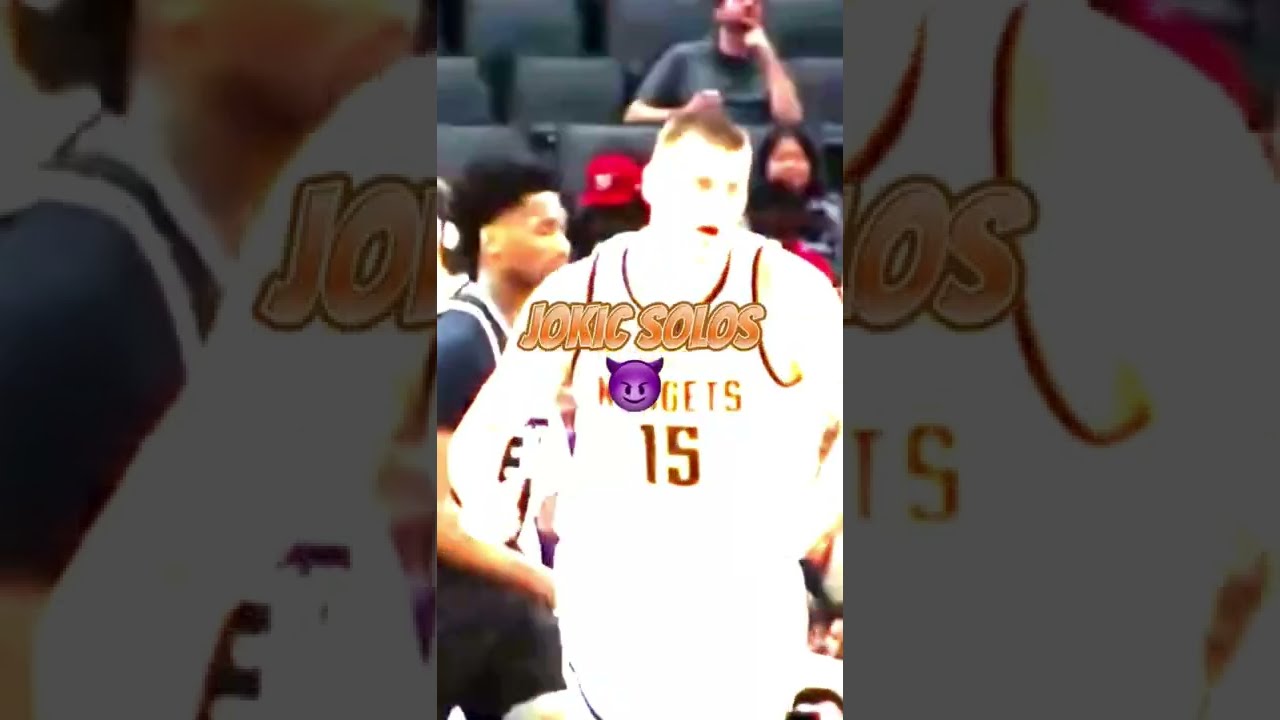The image is a horizontally rectangular, low-quality full-color photograph, divided into three panels. The central panel is overly bright, almost completely washing out the details of the subject, who is a basketball player focused upon in the photograph. This player is wearing a jersey numbered 15 for the Denver Nuggets, and the name "JOKIC" is prominently displayed in orange all-cap letters across the front. Below his name is a small purple horned devil emoji. The player's hairstyle is a crew cut, with some descriptions suggesting a mohawk-like appearance with shaved sides. The image captures him from the waist up. In the background, there are spectators seated in bleachers and another basketball player with short black hair, wearing a blue jersey with a white stripe, walking behind him. The left and right panels of the image are duplicates of the central photograph. If the central panel were removed, the remaining parts would form a complete, albeit larger, version of the same image.